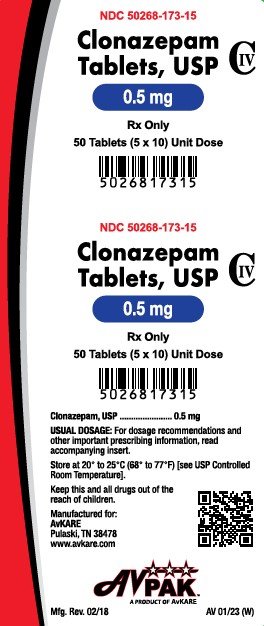The image features a background with multiple colors layered in a non-linear pattern. On the left-hand side, there are distinct layers of color: red, black, and gray, transitioning to a predominantly white background. In the top right corner, a small section of green is visible, as well as a tiny speck of green in the bottom right corner.

Prominently displayed at the top of the image in red, bold, capital letters is the following code: "NDC 50268-173-15." Below it, in black text, is the word "CLONAZEPAM." The next line reads, "tablished, USP," with a capital "C" next to it containing a capital "IV."

Further down, a blue oval with white text prominently displays "0.5 MG." Beneath this, also in black text, is "RX only." Following this, the text reads "50 tablets (5X10)," indicating the packaging format, and "UNIT DOSE" in capital letters.

Below this information is a black and white barcode, with the number sequence "5026817315" printed underneath in black text.

The lower part of the image mirrors the upper part, reiterating the same details: "NDC 50268-173-15" in red, the word "CLONAZEPAM," followed by "tablished, USP," then the capital "C" with a capital "IV," the blue oval with "0.5 MG," "RX only," "50 tablets (5X10)," and "UNIT DOSE." The same barcode and number sequence "5026817315" appears again at the bottom.